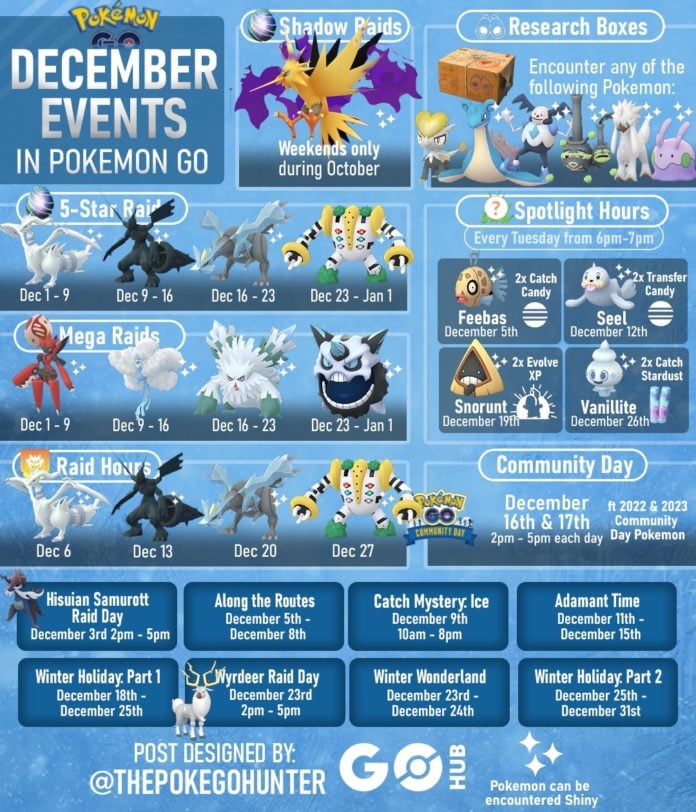The advertisement screenshot features a light blue background adorned with snowflake-like inclusions that convey a wintry theme. In the upper left corner, a darker blue square prominently displays the "Pokémon GO" logo in a stylized yellow font for "Pokémon" and black for "GO." Below this, white text announces, "December events in Pokémon GO."

Moving to the right, a white font box indicates, "Shadow Raids, weekends only during October," with an image of a yellow bird Pokémon centrally positioned within. Adjacent to this, a rectangle highlights "Research Boxes" at the top, followed by white text stating, "Encounter any of the following Pokémon," accompanied by images of five unspecified Pokémon characters.

Beneath this section, the advertisement lists "Five Star Raid," "Mega Raids," and "Raid Hours," each illustrated with different Pokémon images and specific dates, such as "December 1-9." On the far right side, a notice reads, "Spotlight Hours," specifying that these events occur every Tuesday from 6 p.m. to 7 p.m.